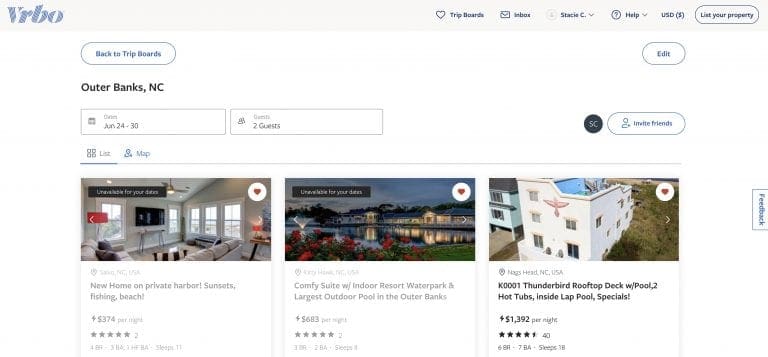On the left side of the image, the VRBO logo is prominently displayed in gray. To the right, various menu options are listed including "Trip Boards," "Inbox," "Help," and an account name that appears to be "Stacey." Additional menu items include a dropdown for assistance and an option labeled "AOSD" with "dollars" in parentheses next to it, likely related to currency settings or bookings. There’s also a feature for listing a property. All of these elements are in black, though the resolution of the website is quite poor, making the text difficult to read.

At the top left corner, there is a button labeled "Back to Trip Boards." Below this, "Outer Banks, NC" is displayed, indicating the location being searched. A date field specifies the trip duration from June 24 through June 30. The search parameters indicate that the booking is for two guests. Below these details, options to view the listings as a list or on a map are provided.

Three property listings are shown: 
1. "New House, New Home on Private Harbor: Sunsets, Fishing, Beach" priced at $374 per night.
2. "Comfy Suite with Indoor Resort Water Park and Largest Outdoor Pool in the Outer Banks" priced at $683 per night.

Underneath the listings, buttons for inviting friends and editing the search parameters are available.